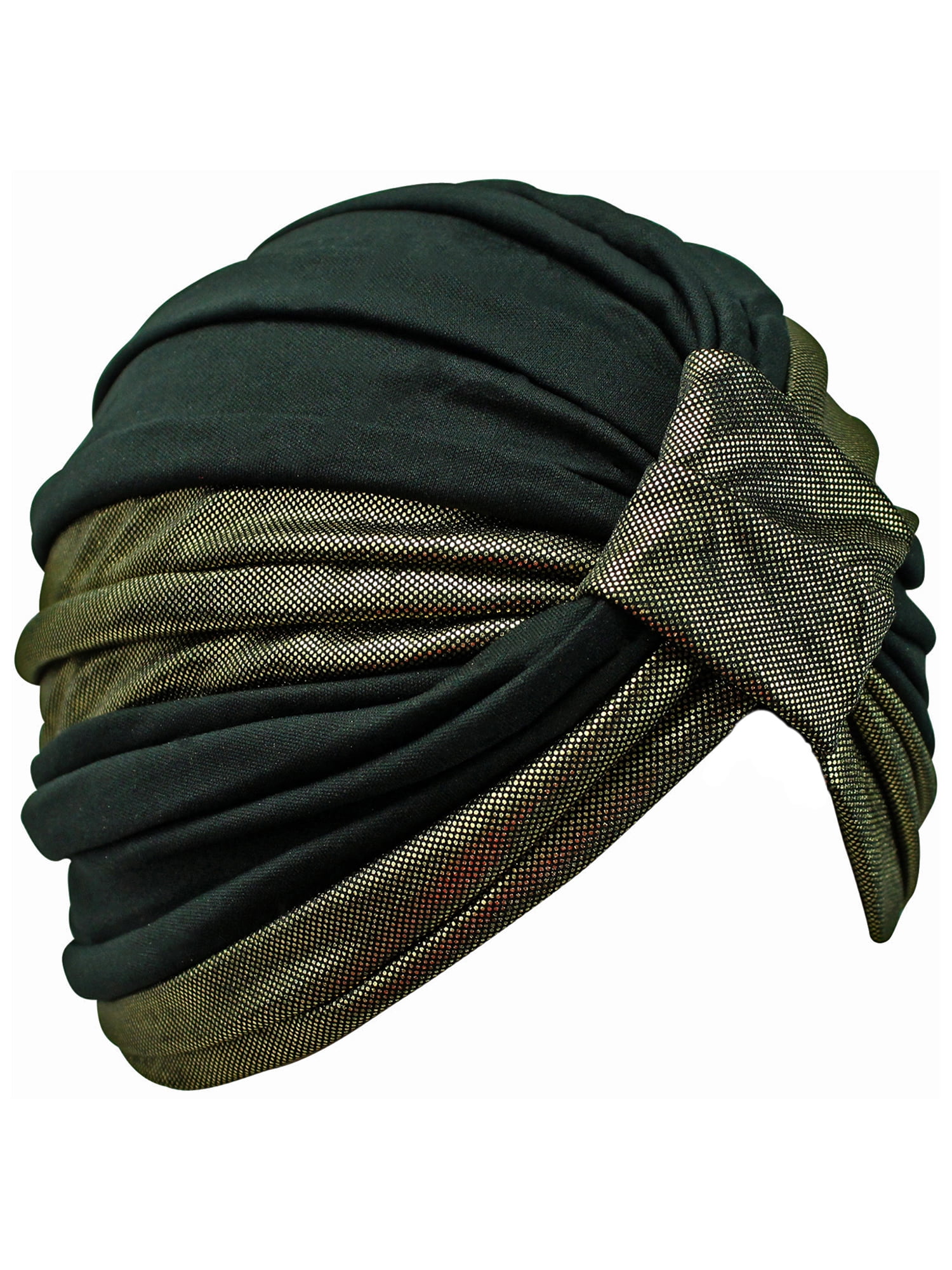The image features an intricate headpiece that resembles a combination of a head and a face mask, possibly inspired by a turban or jousting headgear. The item is crafted entirely from cloth, showcasing a blend of black and shimmering golden-dotted fabric. The primary structure, meant to cover the head, is made of thick, heavy cloth in a deep black color. This black fabric appears bundled and layered, giving a textured, bulky appearance.

The face mask section faces left and is composed of multiple folded layers of cloth. The upper portion of this section boasts a distinctive golden-dotted pattern, followed by a band of folded black cloth in the middle, creating a layered effect. This golden-dotted pattern reappears along the jawline and ear areas, enhancing the decorative design.

At the back of the headpiece, black cloth extends outward, interwoven with sections of the golden-dotted fabric that descend from the ear area. This elaborate design suggests a blend of aesthetic appeal and potential historical or cultural significance.